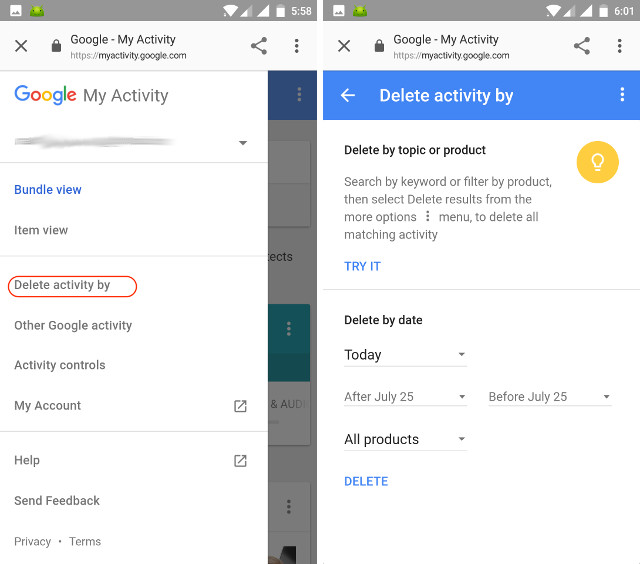This image is a screen capture of two different phone screens displayed side-by-side, both showcasing the user’s interaction with the Google My Activity page. 

**Left Screen:**
- The phone displays the battery icon indicating a nearly full charge, and the time is 5:58. 
- In the upper left-hand corner, signal indicators for two cellular connections and a Wi-Fi connection are visible.
- The screen is titled "Google My Activity," with the URL "https://myactivity.google.com" displayed beneath it.
- The top of the screen has navigation options, including an 'X' button on the upper left and a share icon and a drop-down menu button on the upper right.
- A sidebar menu is prominently displayed, covering most of the screen. The account name is blurred out for privacy.
- Menu options include "Bundle view" (highlighted in blue), "Item view," and "Delete activity by" (circled in red), followed by "Other Google activity," "Activity controls," "My account," "Help," and "Send feedback."

**Right Screen:**
- This screen is on a different part of the Google My Activity interface.
- The section displayed is titled "Delete activity by."
- Instructions listed include "Delete by topic or product," "Search by keyword or filter by product," and "Select delete results from the more options menu to delete all matching activity."

This detailed screen capture highlights the various functionalities and navigation options available within the Google My Activity interface, providing a comprehensive overview of how one can manage and delete their activity data.